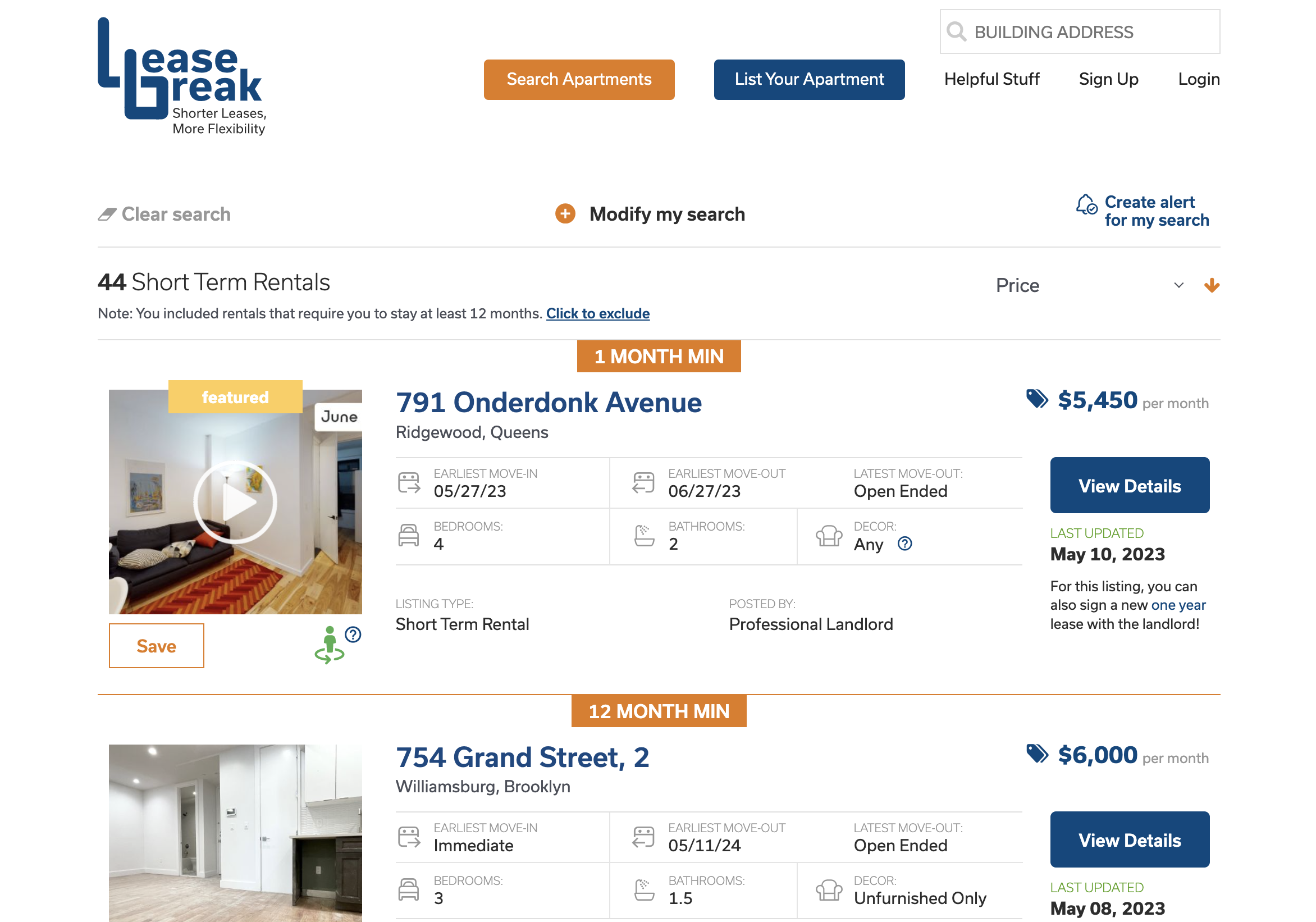The image is a screenshot of an apartment listing website that specializes in short-term rentals, known as Lease Freak. At the top, the website's logo features prominently, with the tagline "Shorter Leases, More Flexibility" beneath it. To the right of the logo are two Call-To-Action (CTA) buttons: an orange one labeled "Surge Apartments" and a blue one titled "List Your Apartment." Adjacent to these buttons, the menu includes additional items—"Helpful Stuff," "Sign Up," and "Log In"—along with a search function box labeled "Building Address" positioned slightly above.

Below the header, the main section showcases a search interface for various short-term rentals. The topmost row features options to "Clear Search," "Modify My Search" in the center, and "Clear Alert for My Search" on the right. Just below, the page title reads "44 Short-Term Rentals," with a note indicating that the listings include rentals requiring a minimum stay of 12 months, with an option to exclude these. On the right side, a sorting function is visible, currently set to organize listings by price.

The page displays two rental listings. Each listing has an image to the left, followed by detailed information on the right. This information includes the apartment address, location, and various details such as "Earliest Move In," "Earliest Move Out," "Latest Move Out," "Bedrooms," "Bathrooms," "Decor," "Listing Type," and "Posted By." To the far right, a blue CTA button labeled "View Details" allows users to access more information. Additionally, the monthly rental price and the date when the listing was last updated are provided.